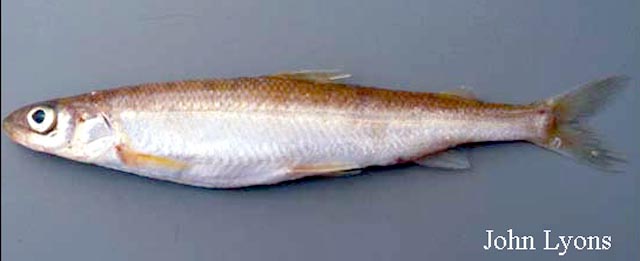This color photograph features a long, slender fish, positioned on a gray surface, and oriented with its head facing to the left. The fish exhibits an angular body with a rust-orange top that transitions into a silver-white middle and underbelly. Its large black-centered eye stands out prominently. The fish has translucent yellow fins: one on the top, two on the sides close to its body, and pointed tail fins. The fish's small mouth and gills are closed, adding to its streamlined appearance. The name "John Lyons" is discreetly placed in the bottom right corner of the image.